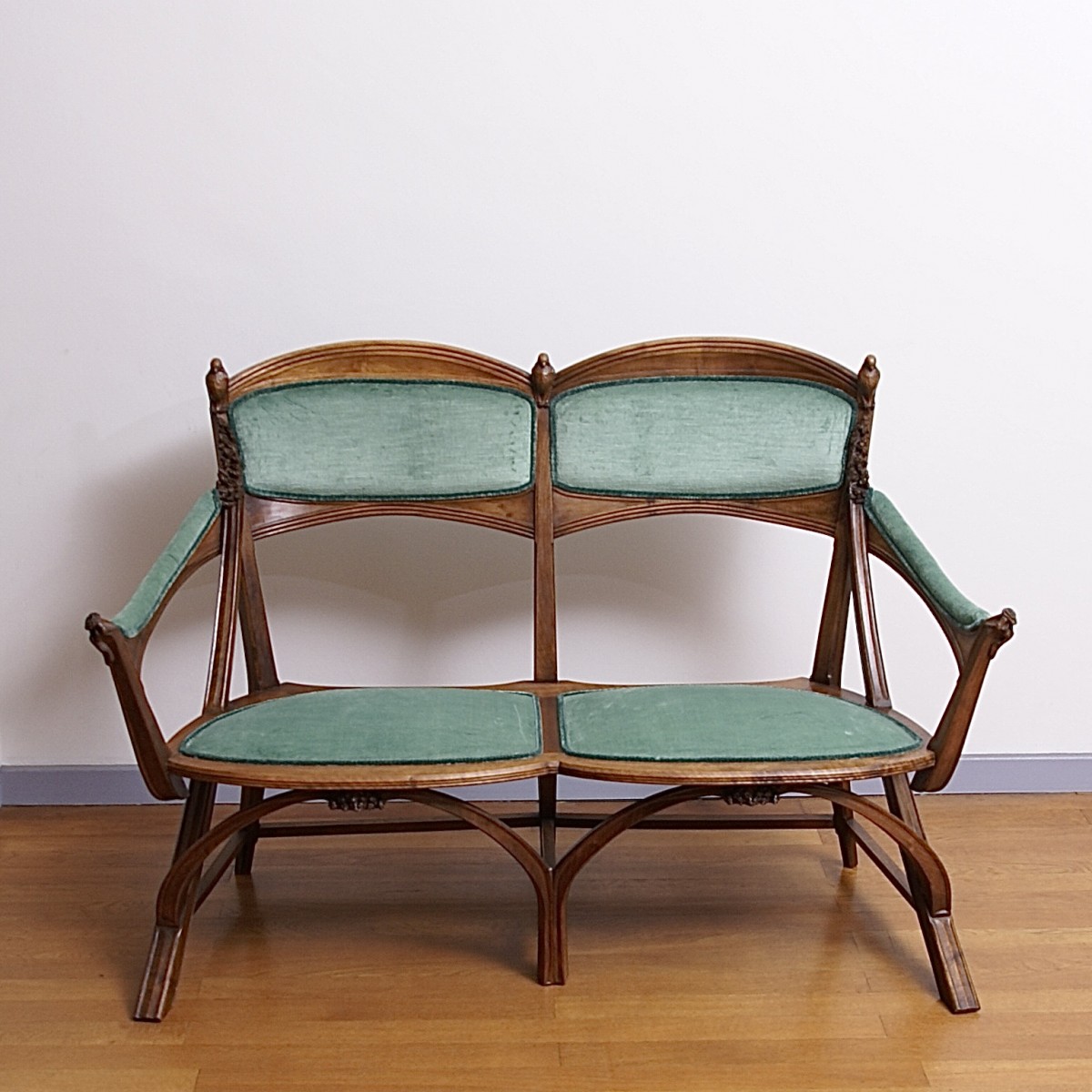The image depicts an intricately designed wooden tandem chair, crafted from dark wood. This double-seater chair features individual armrests on either side but lacks a center armrest, creating distinct seating areas for two people. Each seat is upholstered with green velvet cushions, which also extend to the backrests and armrests, providing comfort while clearly partitioning the seating spaces. The chair is adorned with detailed carvings, particularly noticeable on the backrests and beneath the seats, giving it a vintage aesthetic. This elegantly crafted piece is placed on a light wooden floor against a simple white wall. The wall is complemented by a dark gray baseboard that runs along the bottom, adding a subtle contrast to the setting.